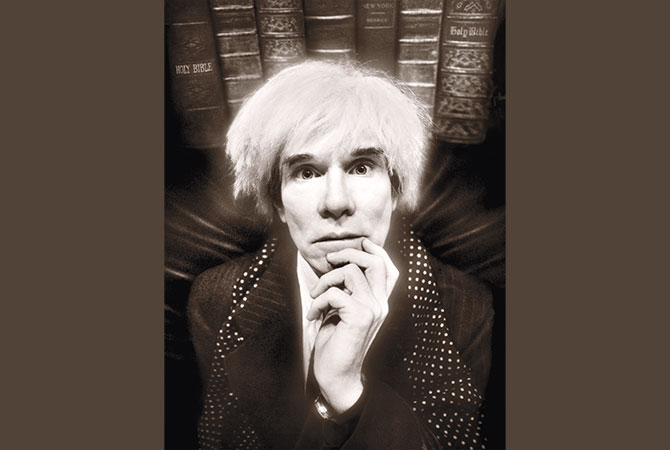In this highly detailed photograph, a gentleman with scraggly, shaggy white hair is seated in a brown chair that matches the dark brown border of the image. The man, captured in a close-up shot, is holding his chin while looking directly into the camera with a concerned expression. His attire includes a pinstripe black suit, adorned with a jeweled collar, and a long polka dot scarf draped around his neck and shoulders. Behind him is a background of ornate, decorative older-style books, including several Bibles with intricate designs on their leather-bound spines. The man has prominent facial features such as thick eyebrows, a wide nose, and very prominent cheekbones. The image is bright and high in contrast, emphasizing the vintage and somewhat dramatic ambiance of the scene.